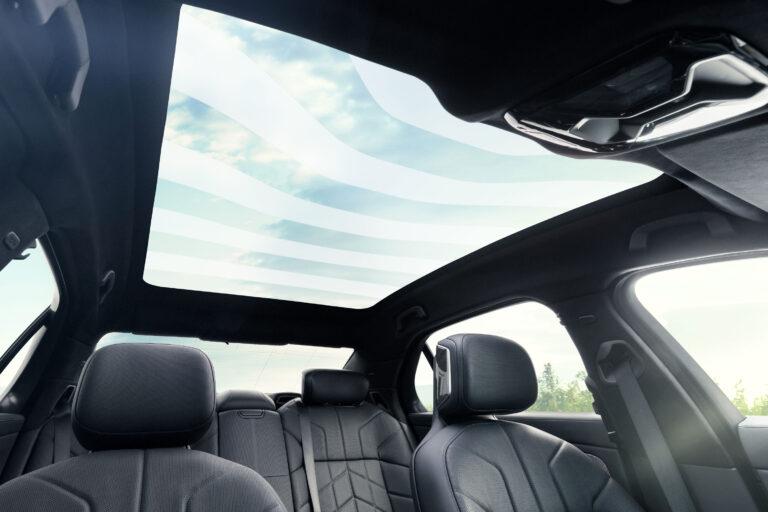The image depicts the interior of a black-trimmed car with a focus on its sunroof. Taken from the passenger seat and angled upwards, the photo captures the entire roof area, including the panoramic sunroof which spans from the front seats to the back. The sunroof is closed and features distinct, horizontally spread white matte lines. The car’s seats are upholstered in a soft, breathable fabric rather than leather, and the front consists of two seats with a potential three-seater row in the back, suggesting this might be an SUV. The interior, including the A-pillars, is entirely black. The backs of the front seats are visible, as well as the seatbelts in their respective areas. The scene outside the car includes trees and sunlight streaming in from the right side, and slight glimpses of a light blue sky with white clouds can be seen through the sunroof. No other passengers are present in the car.